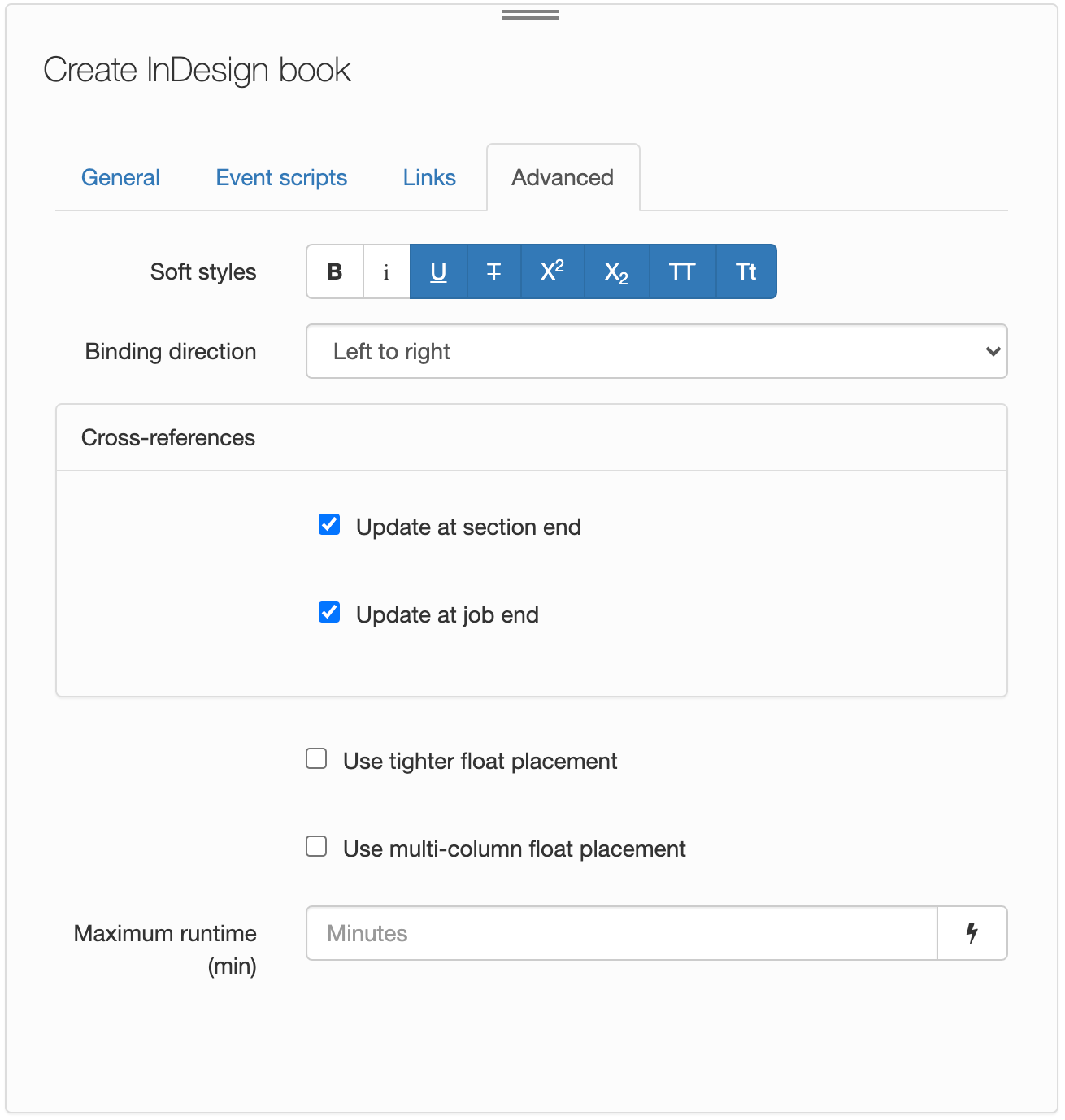This screenshot showcases the settings interface of Adobe InDesign, a prominent desktop publishing software. The interface is primarily set against a white background, with two horizontal dark gray bars positioned centrally. 

At the top of the interface, below the gray bars, the text "Create InDesign Book" is prominently displayed in black font. The settings are divided into several tabs, including "General," "Event Scripts," "Links," and the currently active "Advanced" tab, which is highlighted in black. These tabs are reminiscent of a filing system, visually differentiated by a small underline.

Within the "Advanced" tab, various options are available. In black font, the text highlights "Soft Styles" followed by several formatting icons: a bold "B," an italicized "i," and a series of blue squares containing icons such as an underlined "U," a struck-through "T," a superscript "X²," a subscript "X₂," and a pair of "T" icons indicating small caps and mixed case styles.

Further down, there is a dropdown menu labeled "Binding Direction," currently set to "Left to Right." Below this, there are two checked boxes for options "Update Section End" and "Update Job End." Two additional, unchecked boxes offer the choices "Use Tighter Float Placement" and "Use Multi-Column Float Placement."

At the bottom of the interface, there is a field labeled "Maximum Run Time" with a unit set to minutes, accompanied by a small lightning bolt icon, likely representing a quick action or advanced setting. This detailed interface allows users to finely tune the parameters of their InDesign projects, ensuring precise control over document formatting and behavior.